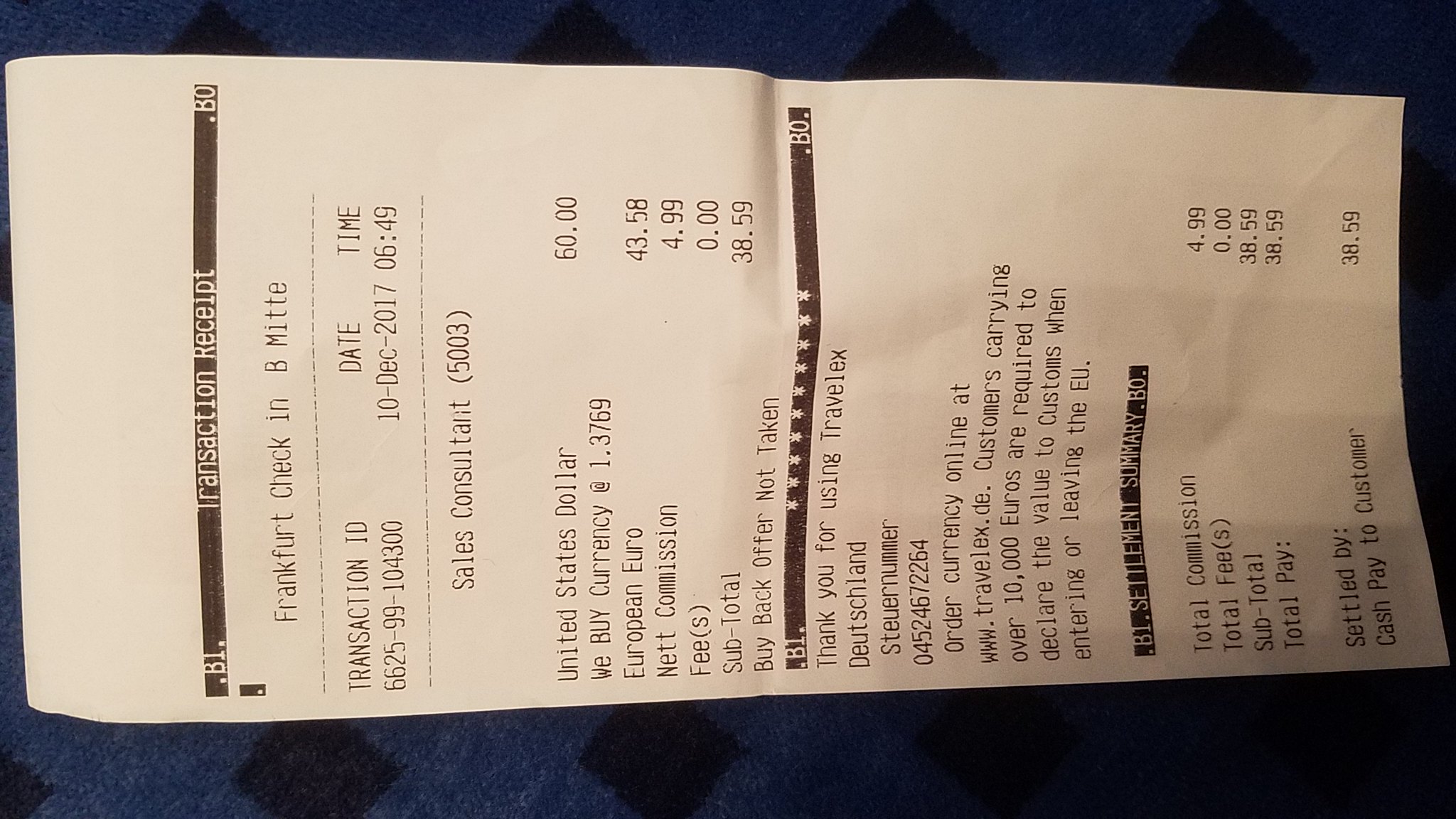This is an image of a transaction receipt from Frankfurt Check-in B, MITTE, photographed lying sideways against a partially shadowed background with a blue carpet featuring dark blue or black diamond shapes. The receipt details a currency exchange transaction dated December 10th, 2017, at 6:49. Issued by sales consultant number 5003, the receipt shows an exchange of $60 USD to €43.58 EUR, with a buy rate of 1.3769. The net commission is listed as $4.99, with no additional fees, bringing the subtotal to $38.59. The receipt also mentions that the buyback offer was not taken. There is a prominent black line separating sections of the receipt. At the bottom, it reads, "Thank you for using Travelex Deutschland," followed by instructions for online orders, and a note on customs declaration for values over €10,000. The receipt is black and white, and concludes with a summary citing a total commission of $4.99, total fees of $0, and a total payout of $38.59, settled by cash.